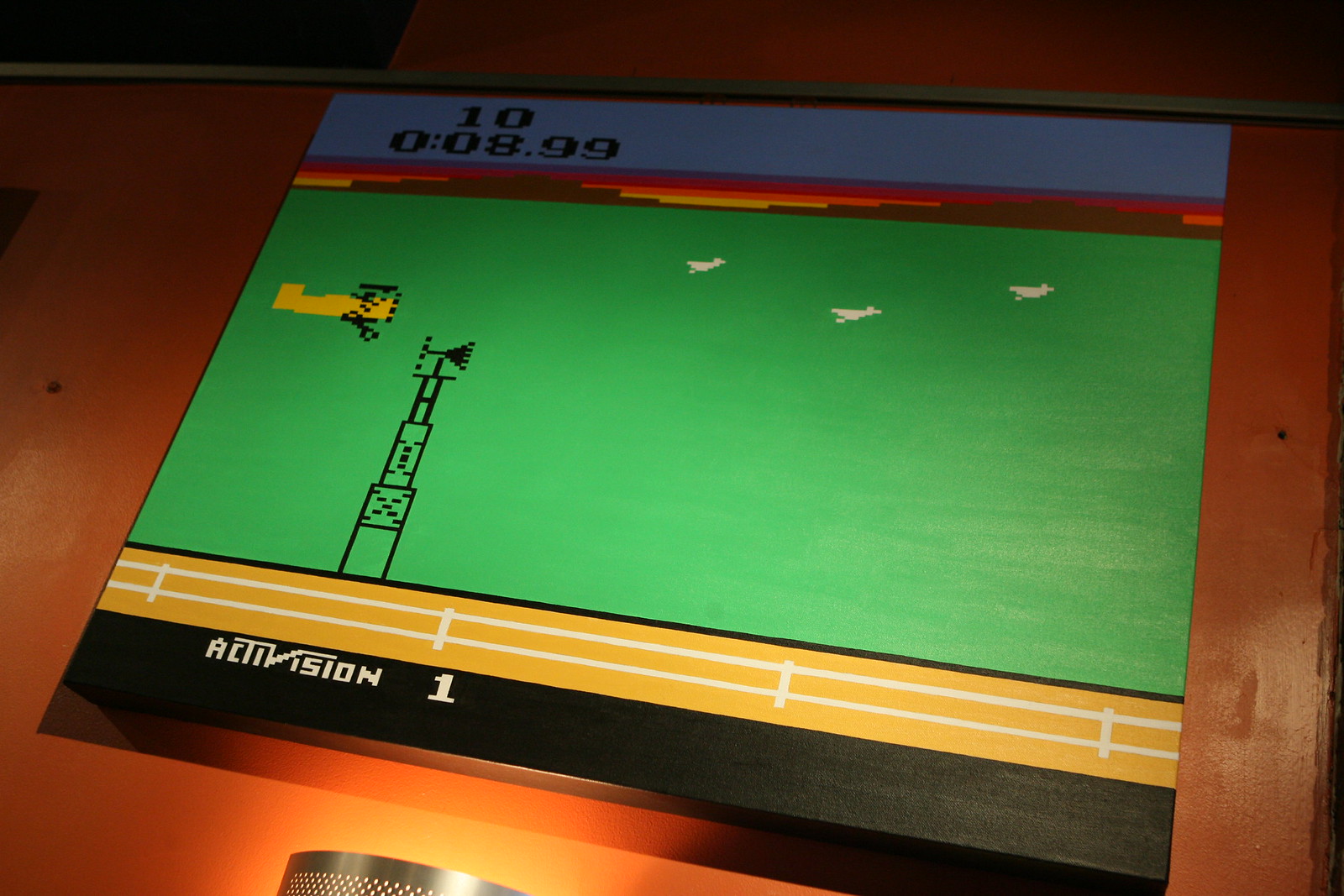The image is a color photograph taken at a slight angle of a computer monitor displaying a vintage video game, identified as an Activision title. The screen tilts slightly to the right, housed within a wooden panel, possibly part of a desk or wall mount. The game features a predominantly green background with a pixelated yellow biplane flying from left to right. The biplane is clearing a rudimentary pixelated communication tower or wind vane structure, while pixelated white birds are visible in the sky above. Below the green field, there is a sandy brown terrain marked by a white fence extending horizontally. In the lower left corner of the screen, the text "Activision 1" is displayed in pixelated lettering. At the top of the screen, various numerical indicators and an alternating red, yellow, and black pattern evoke a timer, adding to the gameplay's vintage aesthetic. The surrounding environment includes a brown wooden table and a hint of light from a nearby fixture, suggesting an indoor setting.